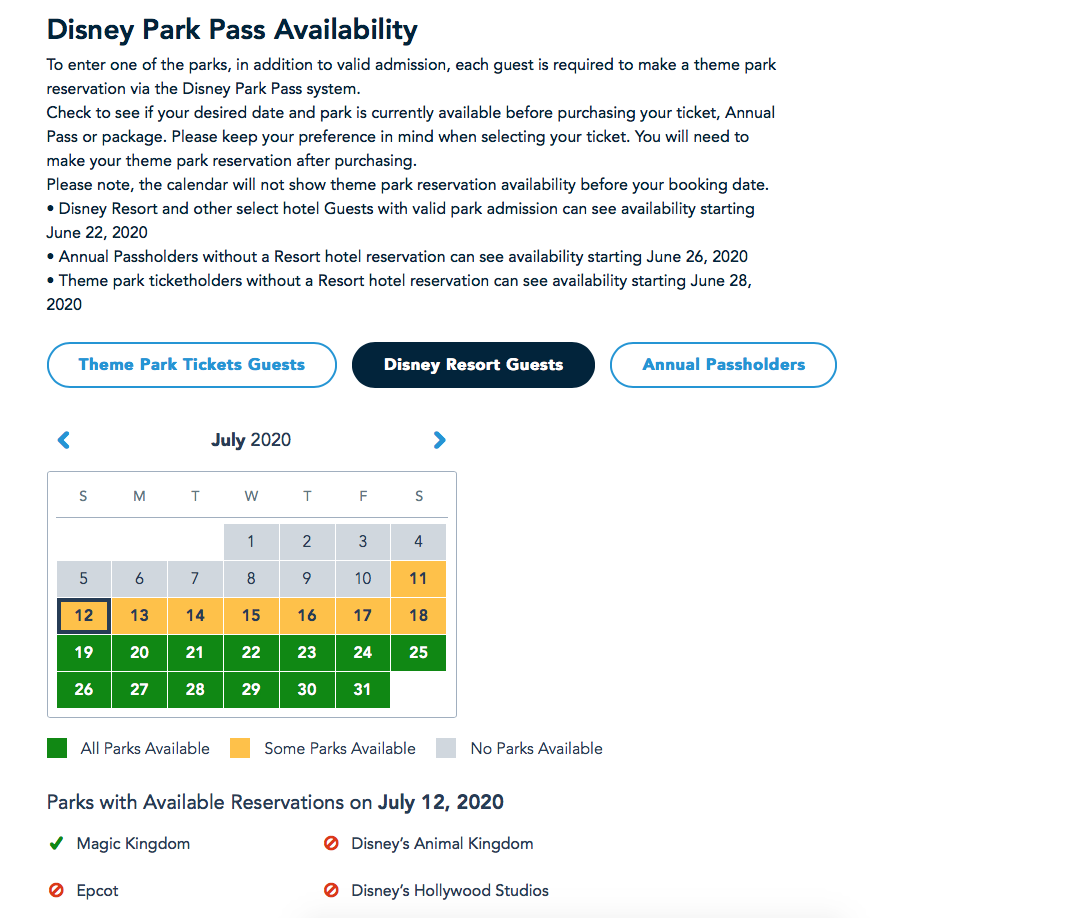To enter one of Disney's parks, each guest is required to have valid admission and make a theme park reservation via the Disney Park Pass system. Before purchasing your ticket, it's important to check if your desired date and park is currently available. 

Guests should keep their preferences in mind, whether they are Annual Pass holders or have booked a package. Reservations cannot be made until after tickets are purchased, and the availability calendar will not display options before the booking date.

- Disney Resort and other Select Hotel Guests with valid park admission can start making reservations on June 22, 2020.
- Annual Pass holders with a resort hotel reservation can begin making reservations on June 26, 2020.
- Theme park ticket holders without a resort hotel reservation can start booking on June 20, 2020.

The reservation system applies every day of the week: Sunday, Monday, Tuesday, Wednesday, Thursday, Friday, and Saturday. Guests are encouraged to make their reservations as soon as possible to secure their preferred dates.